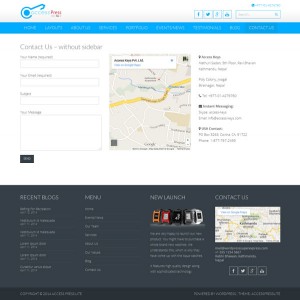The image features a detailed layout, beginning in the upper left corner with a small blue key icon. Just below it, a long blue rectangle, approximately six to seven inches in length, is visible. Centrally, there is a square segment resembling a map, possibly sourced from Google Maps. This map appears distant and small, primarily rendered in light gray with white lines running through it, and it prominently displays a yellow road and black text. 

To the left of the map, the words "Contact Us" are displayed, accompanied by designated fields for entering your name, phone number, and other relevant contact information. The upper right corner showcases options to connect with the company on Facebook, Twitter, and Instagram. 

At the bottom of the image, a large dark gray square provides additional details, including links to the menu, information about new launches, contact options, and recent blogs. This section also features social media sharing options for Facebook, Twitter, and Instagram, with each platform's icon situated in a white square for easy identification.